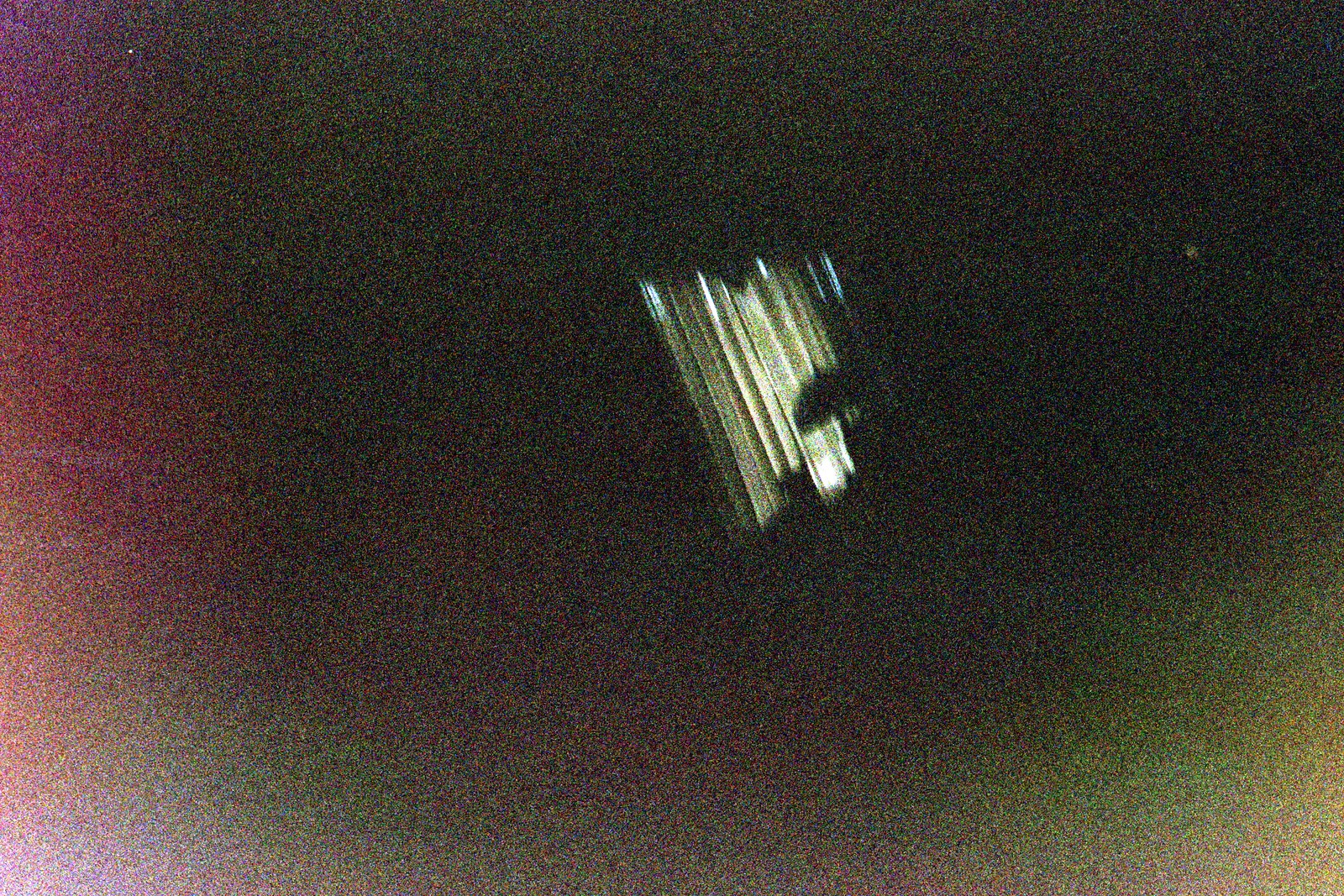This photograph appears to have been taken indoors at night or in an unlit room, resulting in an extremely grainy and fuzzy image. On the left side, there's some white, reflected light illuminating parts of the scene. In the bottom right corner, there are flashes of pink, yellow, and green colors. The focal point of the image is a window positioned at an unusual angle, tilted towards the left. The window is adorned with cream or white curtains, silhouetting a lamp against them, suggesting the photo was taken from inside the room.